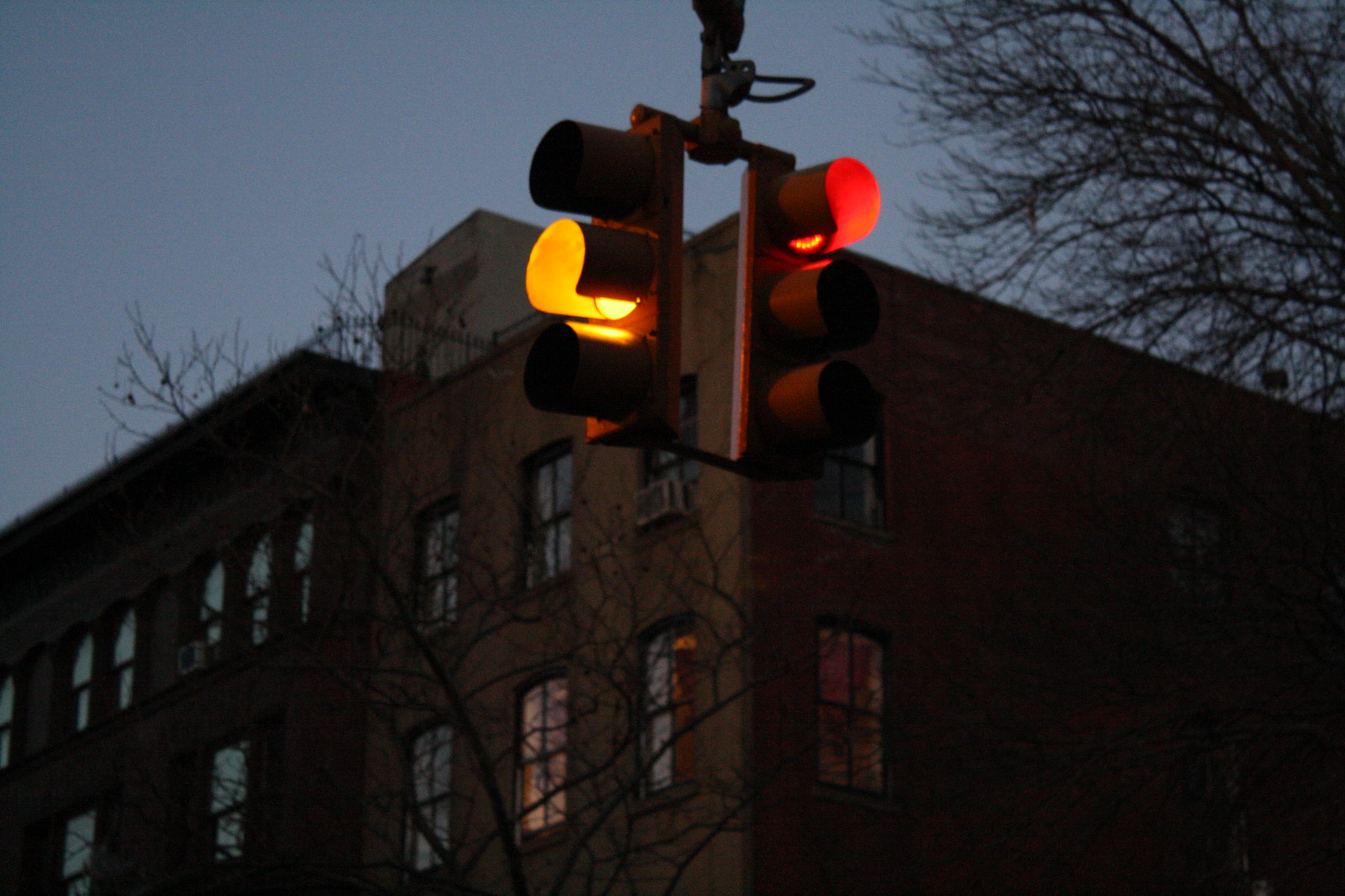This rectangular, landscape-oriented photograph captures a traffic stop signal at dusk. The close-up shot prominently features the signal, which hangs from an unseen post near the top of the image. The signal has two lights: one facing left, displaying a yellow light, and another on the right, perpendicular to the first, glowing red. The sky transitions to a darkening blue, framing the intersection of a dark brown building seen from its corner, with some of its windows softly illuminated from within. Leafless trees appear in the upper right-hand corner and in front of the building, adding to the stark, wintry atmosphere.